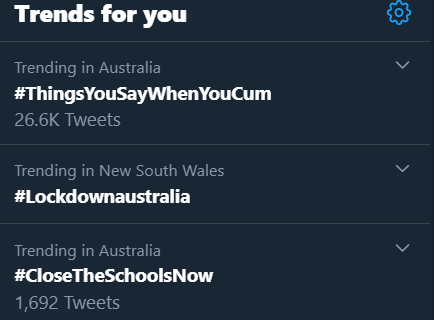The image features a dark blue background with several trending topics displayed in white and grey text. At the top, the heading "Trends for you" is written in bold white text. To its right, there is a blue settings icon depicted as a gear. Below this, in grey text, it reads "Trending in Australia." 

The first trending topic is "#thingsyousaywhenyoucome," which has accumulated 26.6k tweets. Next to this, there is a down arrow icon. Beneath it, another trend is noted in light grey text, stating "Trending in New South Wales," followed by the hashtag "#lockdownAustralia" in bold white text with a white down arrow next to it.

Further down, another trend is highlighted with the phrase "Trending in Australia" in grey text. Directly below, in bold white text, it reads "#closetheschoolsnow," with a grey text note indicating that it has 1,692 tweets. Throughout the image, several thin grey lines create divisions between these topics. The bold white text contrasts sharply with the thinner grey text, enhancing readability and organization.